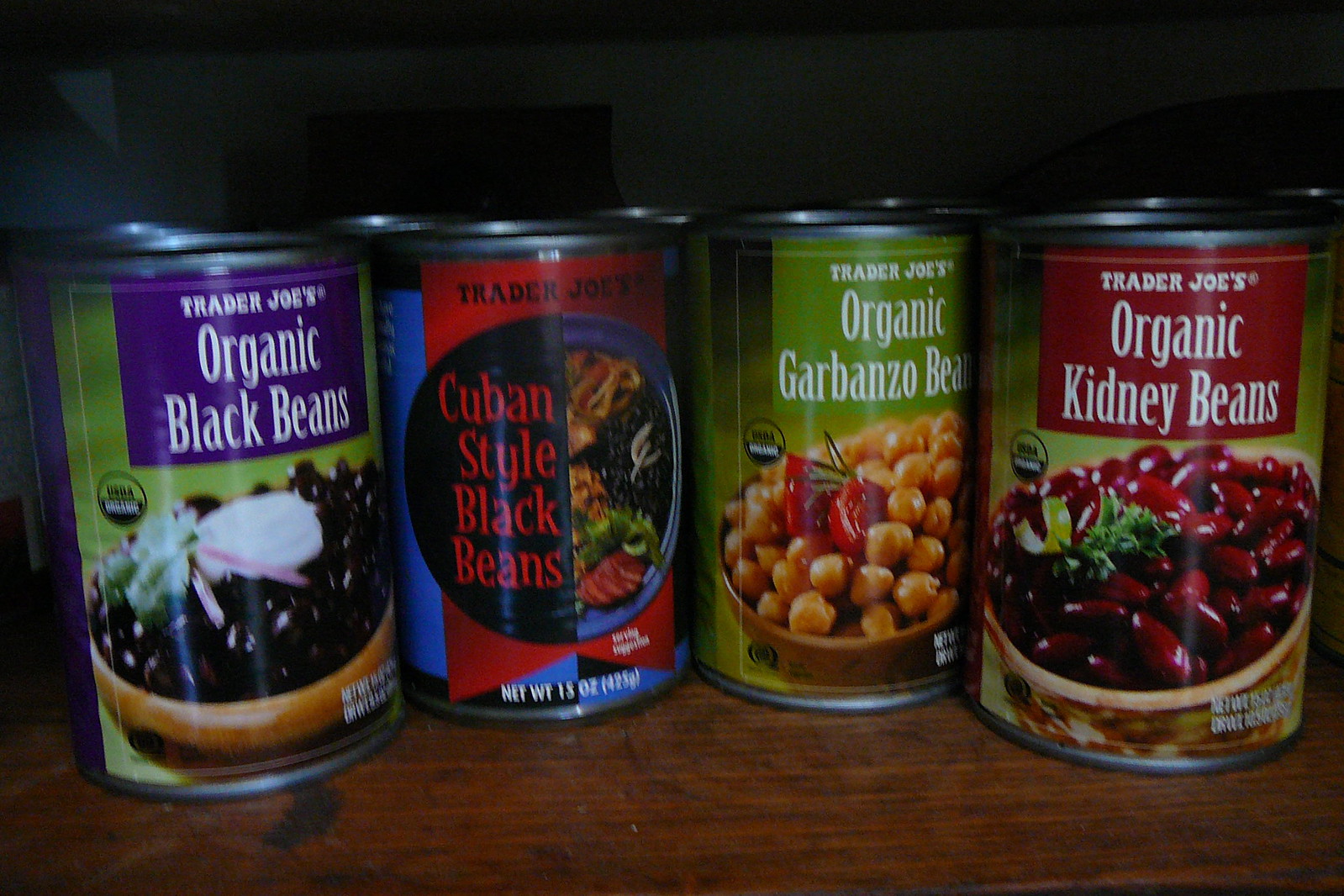This photograph, likely taken in portrait mode, captures four cans of organic beans from Trader Joe's, neatly arranged from left to right on an old, stained wooden surface. The woody texture appears dirty and dingy, adorned with black stains. No humans are present in the image, allowing the focus to solely be on the cans and their surroundings. 

- The first can showcases Trader Joe's Organic Black Beans with a green label accentuated by a vibrant purple rectangle featuring the product name. The label depicts the beans along with pieces of white and red onion, all against a green leafy backdrop.
  
- The second can presents Trader Joe's Cuban Style Black Beans, distinguished by a red and dark blue theme. The label features an image of black beans mixed with what appears to be pork and chicken chunks, framed by colorful triangular patterns.

- The third can displays Trader Joe's Organic Garbanzo Beans, adorned with a predominantly green label. The can’s design includes a lime green rectangle with white text, images of brown garbanzo beans, and slices of red tomatoes accompanied by green leaves.

- The fourth can features Trader Joe's Organic Kidney Beans, encapsulated in a red-themed design with a white-text rectangle. The label shows dark red kidney beans topped with dark and light green garnishes, possibly cilantro and celery.

In the distant background, there is a dark, dimly lit wall that accentuates an ambiance of neglect, further emphasized by a black flat-screen TV situated on the left side. The detailed and artistic can designs contrasted against the worn wooden surface create an intriguing visual dichotomy in this everyday setting.